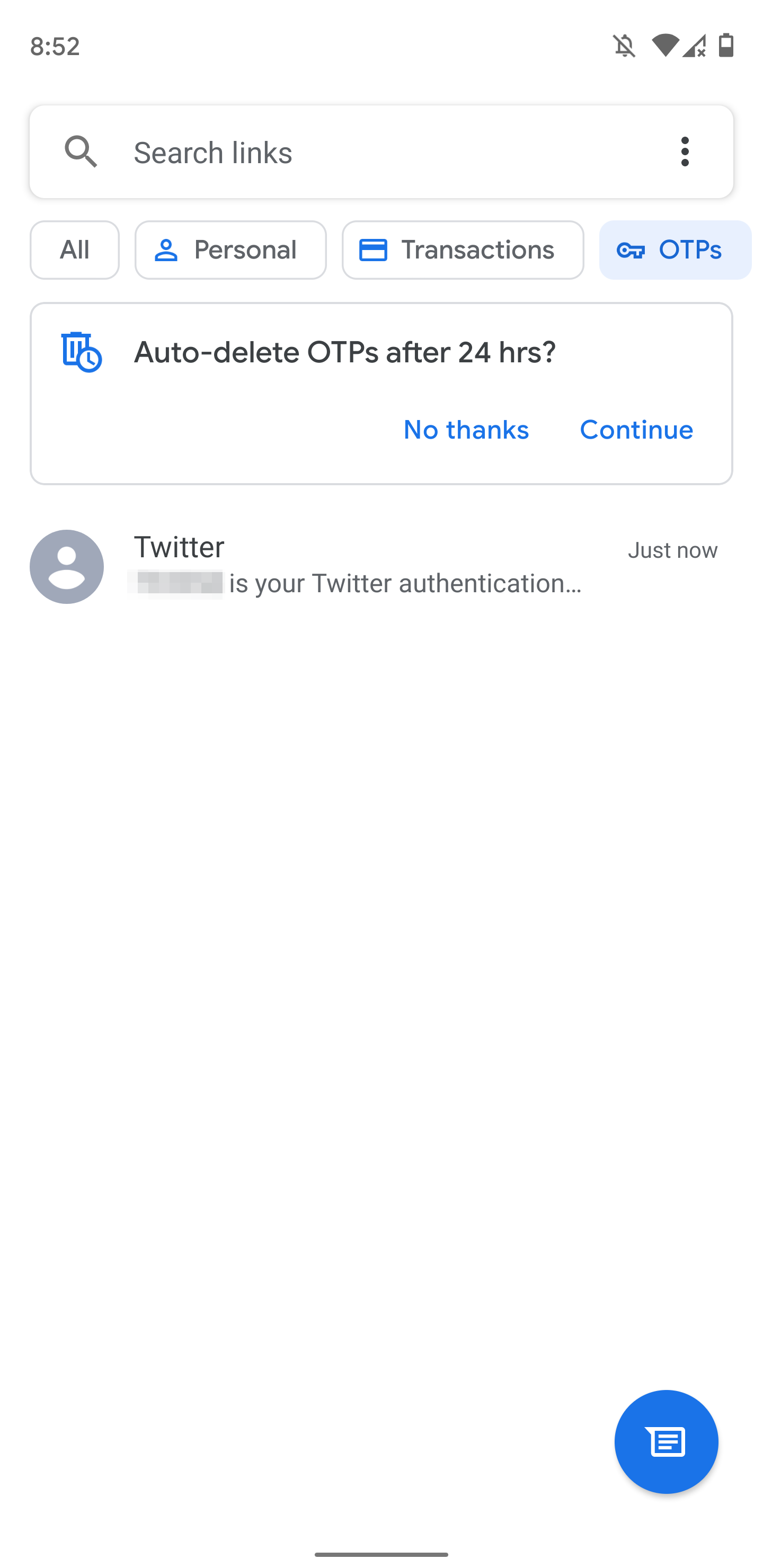This image is a screenshot from a phone displaying a search page from an unidentified app. At the very top left of the screen, the time is shown as 8:52. Directly across to the right, various icons indicate the phone's status: the ringer is off, Wi-Fi is fully connected, there is no cellular service, and the battery is slightly less than half full.

Below the status bar, there is a search box with the placeholder text "Search links." To the left of this box is a magnifying glass icon, and to the right are three vertical dots.

Under the search box are four selection tabs arranged horizontally: "All," "Personal," "Transactions," and "OTPs," with the "OTPs" tab currently highlighted, accompanied by a key icon.

Following these tabs, there is a notification box offering an option to "Auto delete OTPs after 24 hours?" with two buttons below it: "No Thanks" and "Continue."

Beneath this notification box is a circular icon with a generic white silhouette representing a user's profile picture, accompanied by the text "Twitter is your Twitter authentication."

The remainder of the screen is largely blank, occupying more than half of the display. At the very bottom, there is a small scroll bar with a marker at its center. To the right of the scroll bar, a blue circular icon with an image resembling a speech bubble, possibly indicating a chat function, is visible.